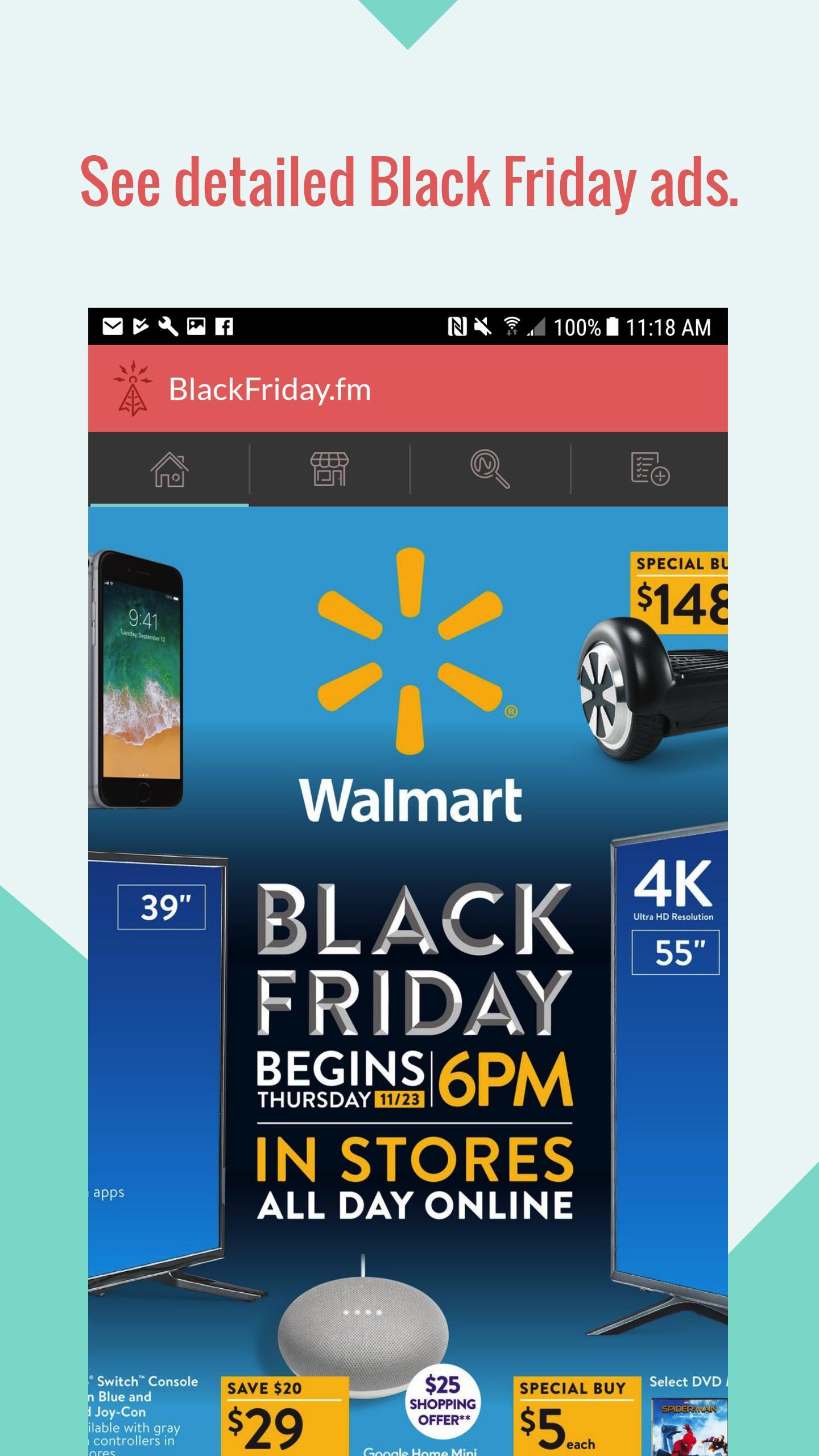This Black Friday advertisement from Walmart features a vibrant and eye-catching design. The ad is framed with a mint green border, which deepens to a darker mint shade at the bottom. Dominating the top of the screen, bold red text announces, "See Detail Black Friday Ads." Below this banner lies the main body of the advertisement.

Set against a blue background, the iconic Walmart sunburst logo is prominently displayed, accompanied by the name "Walmart." The centerpiece message declares, "Black Friday begins Thursday, 11-23 at 6 PM," with "6 PM" highlighted in bright yellow for emphasis. Below this, also in yellow, the text "In stores" is prominently featured, while underneath, in white letters, it states, "All day long."

The central part of the ad showcases two televisions. To the right, a 55-inch 4K TV is highlighted, while on the left, a 39-inch TV is featured. Unfortunately, no prices are visible for these items. 

Towards the bottom of the advertisement, a selection of deals is presented on a dark mint green background. Here, shoppers are informed about "Special Buy" DVDs available for $5, a Nintendo Switch controller priced at $29, and a $25 shopping offer enclosed within a circular graphic.

This detailed and colorful advertisement effectively communicates Walmart's appealing Black Friday deals.